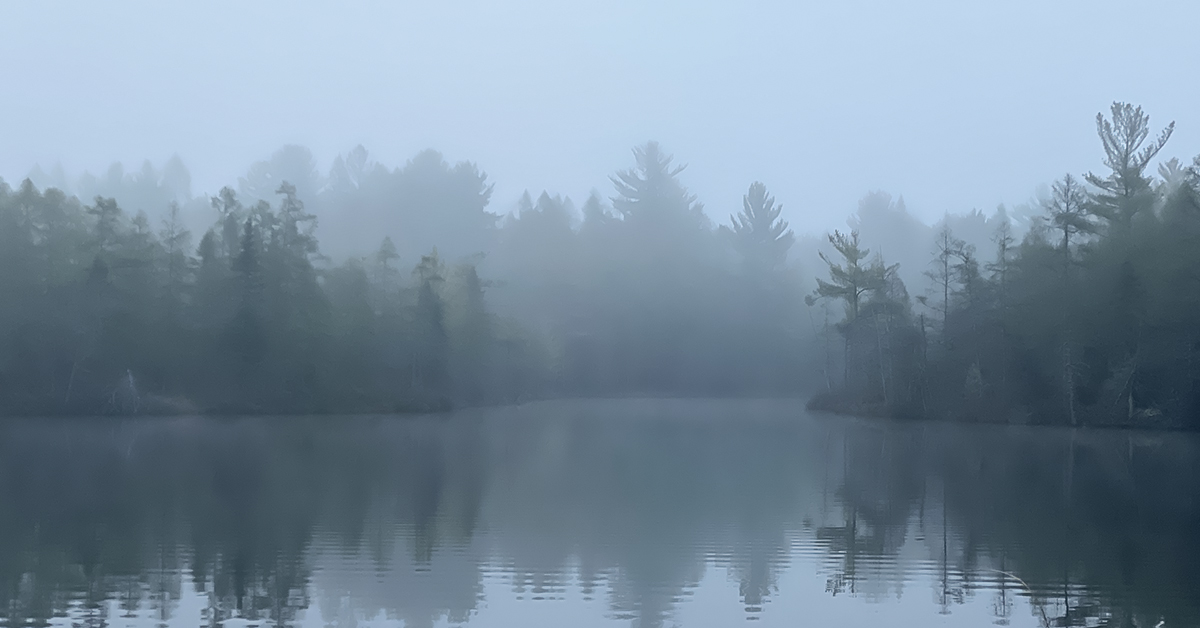The image depicts a serene and foggy natural scene, likely a river, although it could be a lake that leads into a river. The bottom half of the picture is dominated by a reflective body of water, capturing the overhanging trees, which create an almost symmetrical mirroring effect. The water's surface has gentle horizontal ripples indicating movement, and its brownish tint adds to the natural ambiance. Surrounding the water, there is a dense, unbroken line of coniferous trees that appear to spread into the distance. Further back, the trees blend into the fog, creating a misty, cloudy backdrop that enshrouds the entire scene. The sky occupies the top third of the image, contributing to the overall foggy and overcast atmosphere. The water flows inward toward the center of the image, suggesting that the river might be narrowing and possibly detouring to the right. The photo exudes a tranquil, almost painting-like quality due to its atmospheric fog and reflective water surface.